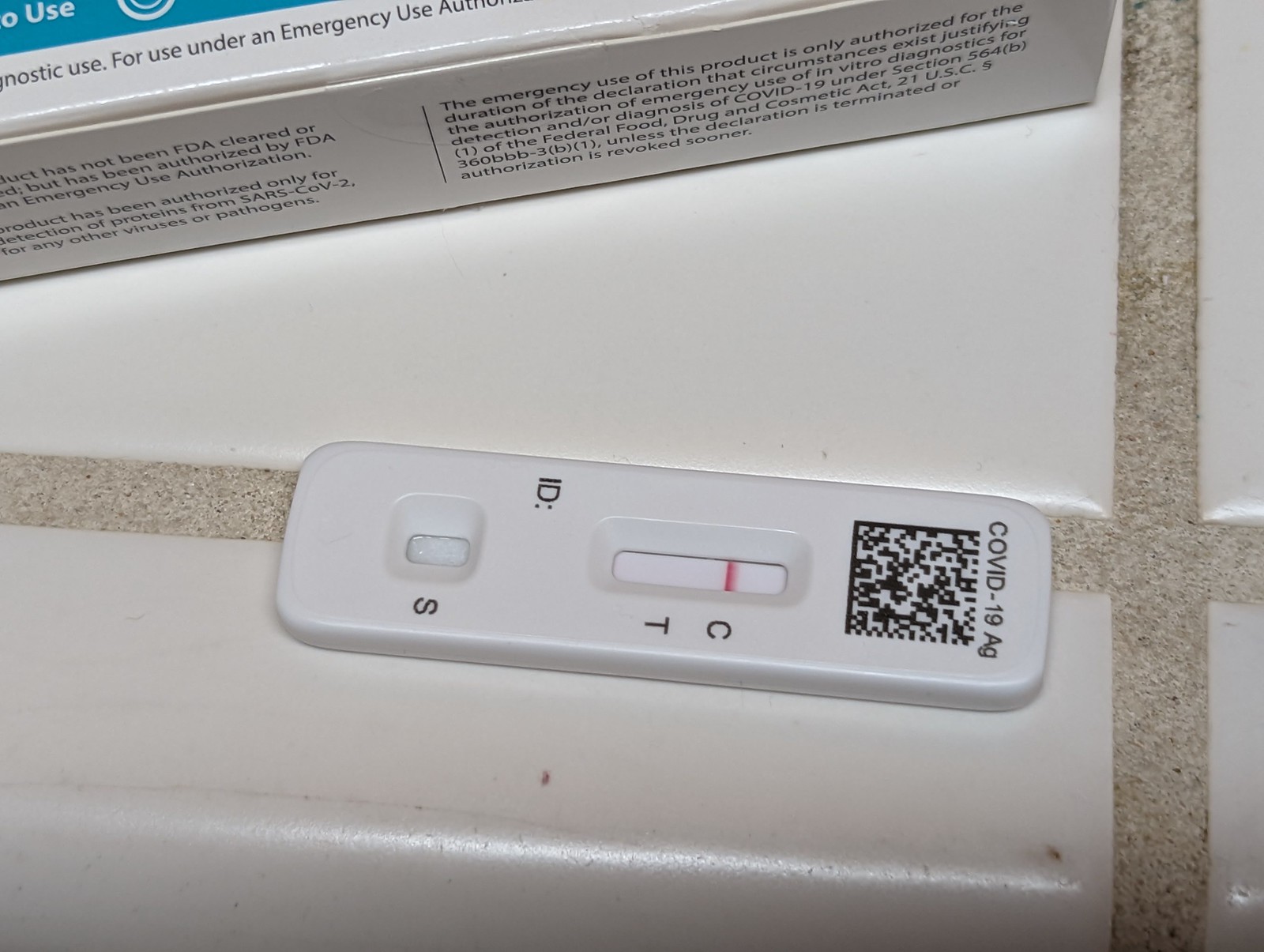The image features a COVID-19 antigen (AG) test. Dominating the background is a prominently white box accented with green, adorned with black lettering. The text on the box indicates that the emergency use of the product is authorized for the duration of the declaration justifying the need for emergency diagnostic tools for COVID-19, in accordance with Section 564 of the Federal Food, Drug, and Cosmetic Act (21 U.S.C. 360bbb-3) unless terminated or revoked earlier.

In the foreground, the COVID-19 test itself is rectangular and compact. One visible section marked with an 'S' features a rectangular opening. Adjacent to it, another segment of the test displays the letters 'T' and 'C,' with a red line next to the 'C.' The term 'ID' is positioned between these two openings at the top. The test's surface includes black dots and symbols on a white background, resembling a scannable QR code.

All these items are placed on white tile flooring. The grout lines between the tiles are a brownish sandy color, adding a subtle contrast to the scene.